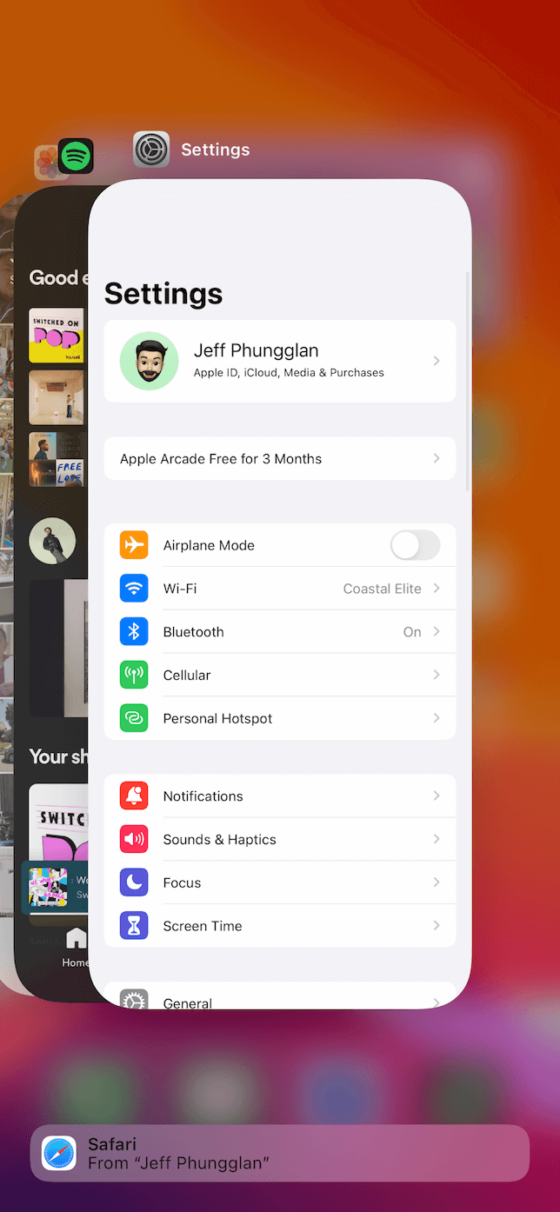The image depicts a smartphone interface overlaid on a background with a gradient from orange at the top to purple at the bottom. In the backdrop, blurred icons resembling those from a typical smartphone home screen add to the depth and thematic connection. At the top of the screen, an orange hue transitions to a purple shade towards the bottom. 

Prominently featured is the settings page of a smartphone under the Apple ID section, attributed to Jeff Phungalan, displaying the Apple ID and various settings options such as "Apple Arcade free for three months," "Airplane mode: Off," "Wi-Fi: Coastal Elite," "Bluetooth: On," along with options for "Cellular and Personal Hotspot," "Notifications," "Sound and Haptics," "Focus," "Screen Time," and "General."

Additionally, at the bottom, a search bar is visible featuring a white and blue compass icon labeled "Safari," indicating Jeff Phungalan as the subscriber. Below this settings page, a black screen section includes a series of icons, with the Spotify logo discernibly placed in the upper left corner.